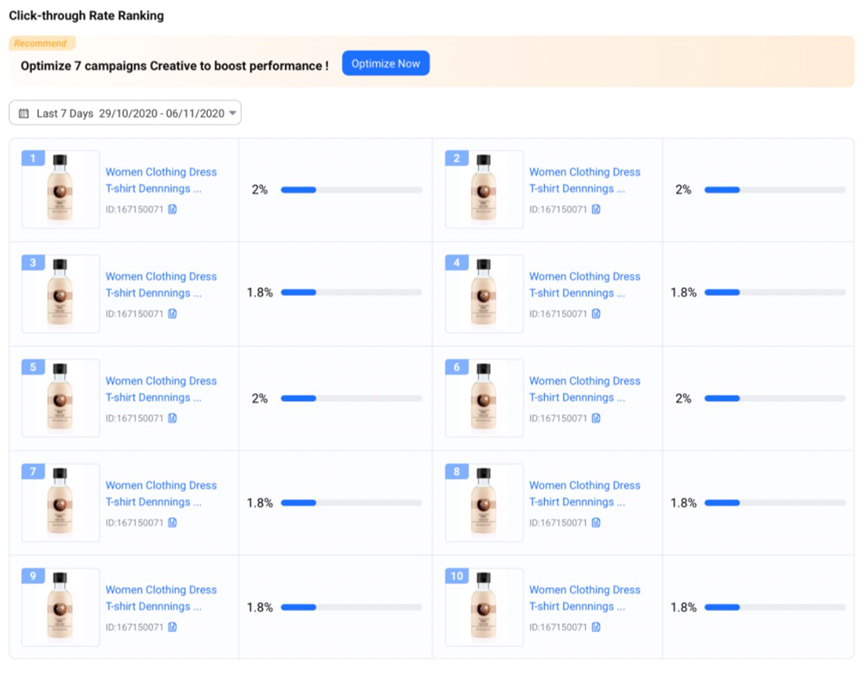The image presented has a white background with various text elements and graphical components. At the top, in prominent black text, it reads "Click Through Rate Ranking." Below this, there is an orange box featuring the text "Recommended." This orange box is nested within a larger pink rectangular box that contains additional text in black: "Optimize seven campaign creative to boost performance."

Adjacent to the pink box is a dark blue, oblong-shaped box that says "Optimize Now" in bold white text. Directly beneath this setup is a drop-down menu displaying the date range "Last 7 Days: 29/10/2020 through 06/11/2020."

The lower section of the image is organized into two columns. On the left, there appears to be what looks like a bottle filled with pink liquid and sealed with a black lid. However, the label next to this image reads "Women's Clothing: Dress, T-Shirt, Jeans" in blue text, which does not match the bottle content depicted. Next to this conflicting label, a percentage is displayed, stating "2%."

This detailed layout appears to be a user interface designed for analyzing and optimizing ad campaign performance metrics.